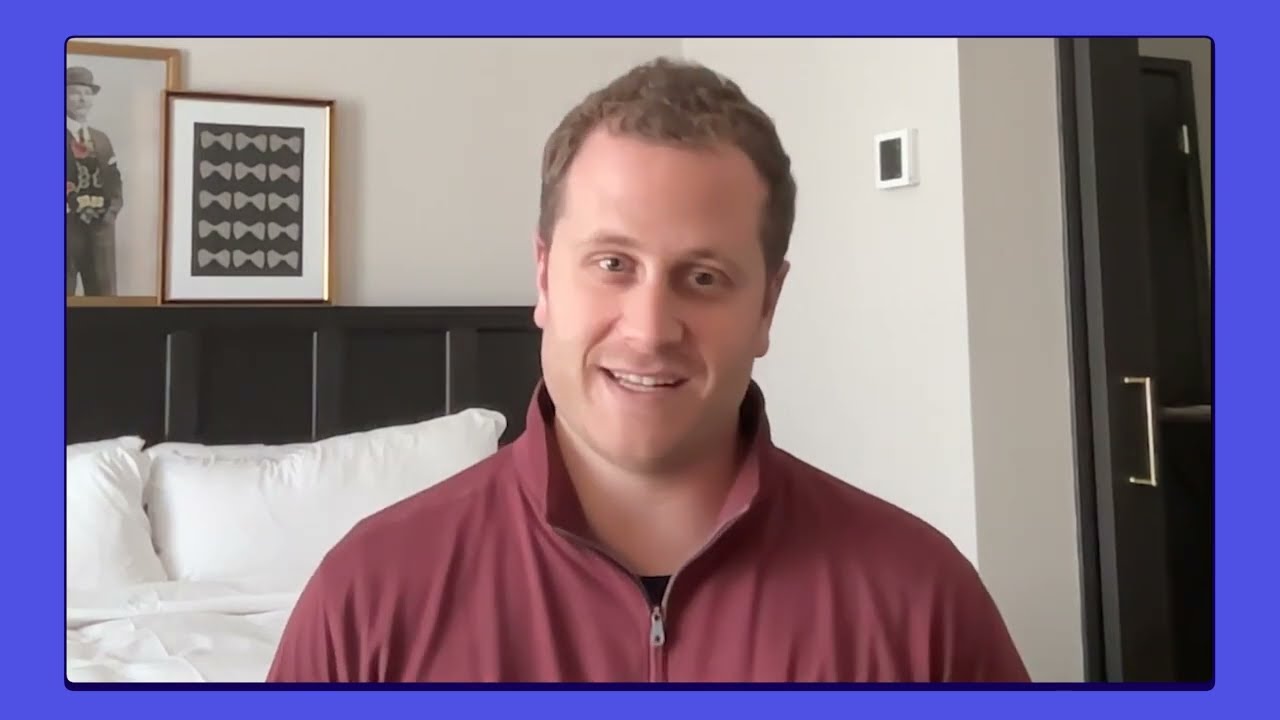In this detailed screenshot from a video call, a white man with short, curly blonde hair and a receding hairline is seen sitting in his bedroom. He is clean-shaven, wearing a zipped-up maroon pullover jacket over what appears to be a black shirt. The room, illuminated by a white wall, features a bed with white sheets, white pillows, and a distinctive black headboard. The background reveals an array of details: a black and white picture of a man, potentially Charlie Chaplin, another frame with rows of bow tie graphics, a thermostat, a brown door with a silver handle, and a mirror. The image is outlined by a blue border, indicative of a Zoom or FaceTime video call context, as the man appears to be talking and slightly smiling into the webcam.